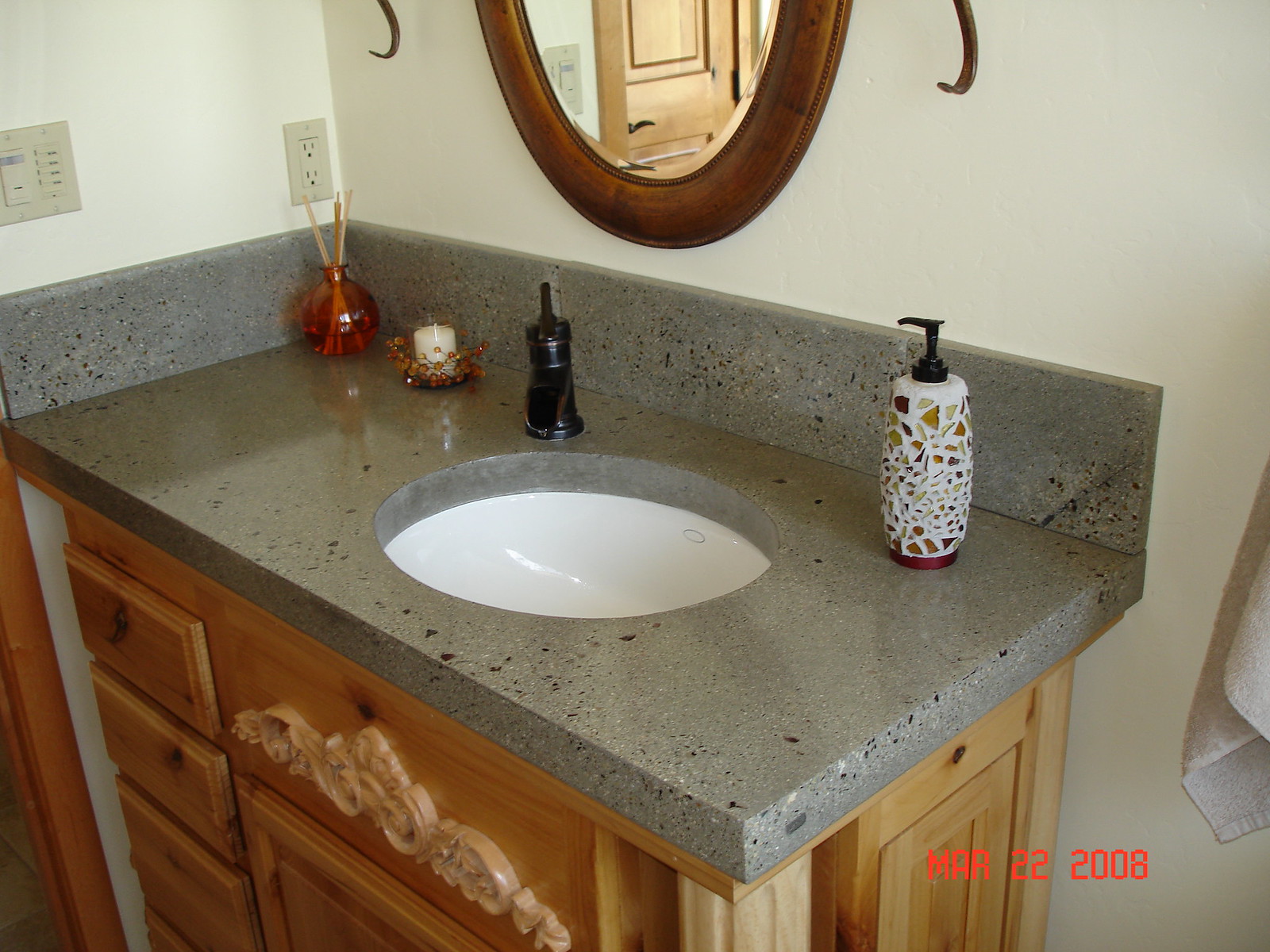This landscape-oriented photograph captures a bathroom sink area with a meticulous attention to detail. The white walls form a sharp corner slightly left of center. Adjacent to the left side of the image, a gray two-plug electrical outlet is visible on the corner of the wall. The sink countertop is crafted from granite with a sophisticated blend of gray and black textures, complemented by a coordinating small black backsplash.

On the countertop, to the left, rests a striking red glass circular container filled with three stick-like objects resembling popsicle sticks. Immediately to the right of it is a small white candle. To the left of the sink, a sleek black faucet adds a modern touch. The soap dispenser, featuring a white background with multicolored accents and topped with a black handle, showcases unique design elements. 

The wooden base of the sink extends to the bottom edge of the photograph, anchoring the scene in warm, earthy tones. An orange and green date stamp, "March 22, 2008," is positioned at the bottom right corner, adding a nostalgic timestamp. Completing the image, the top shows a half cut-off oval mirror framed in dark brown wood, enhancing the bathroom's elegant aesthetic.